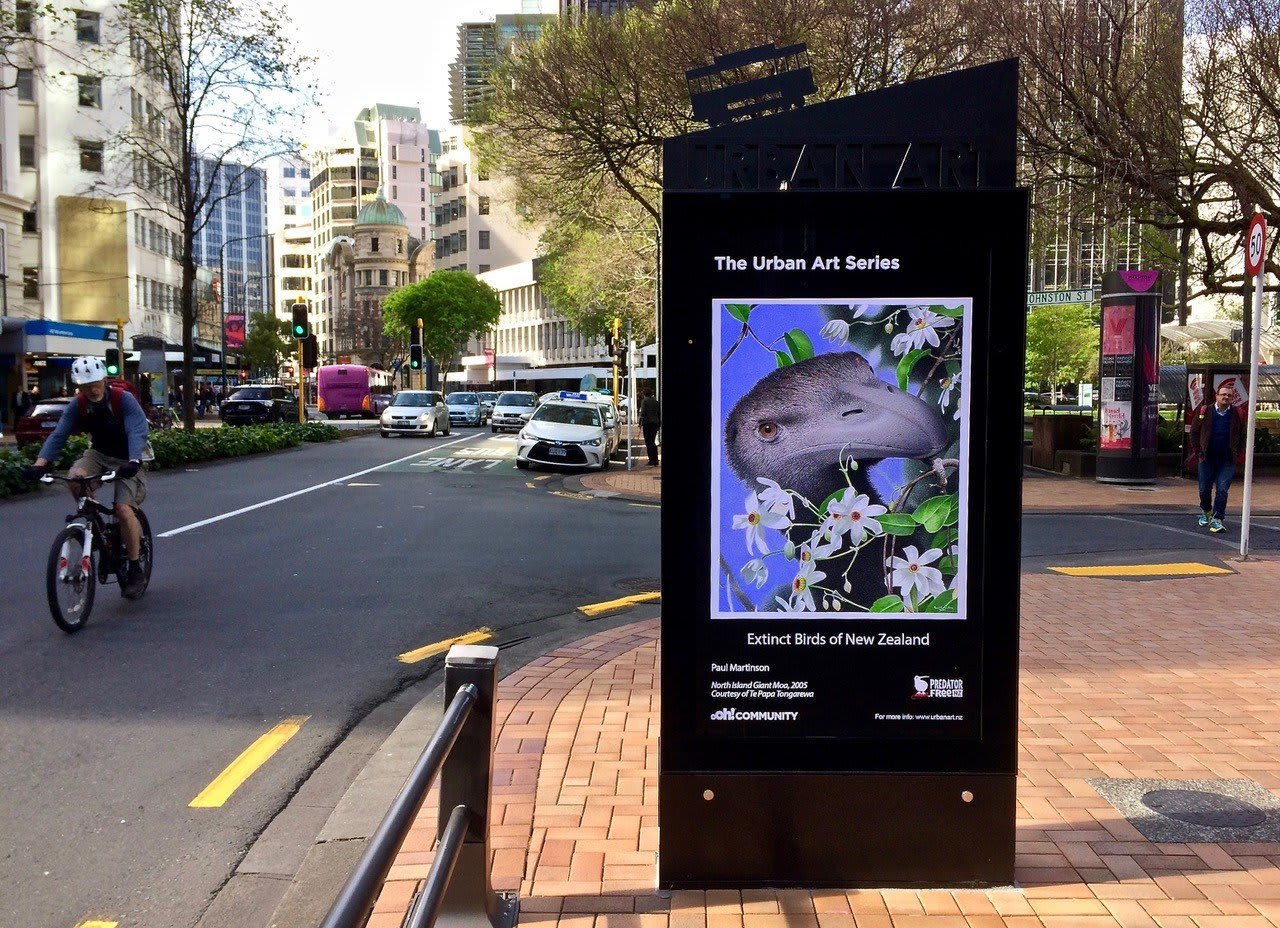The image captures a bustling city street, likely in Europe, featuring Johnston Street. The scene includes a variety of elements such as moving traffic, parked cars, and several pedestrians - one walking and another riding a bicycle with a helmet. Distinctive road signage, including a European-style speed limit sign indicating 50 in a white circle with a red border, enhances the urban atmosphere.

A dominant feature in the center of the image is a tall, black kiosk or sign with an angled top. This sign serves as an advertisement for an art exhibit titled "The Urban Art Series: Extinct Birds of New Zealand." The poster on the sign showcases a detailed, illustrated bird with a large beak, surrounded by white flowers and green foliage set against a blue sky. Below the main title is additional, smaller text that is not fully legible but indicates it's an art series. Surrounding the street are high-rise buildings, adding to the metropolitan vibe of the photograph.